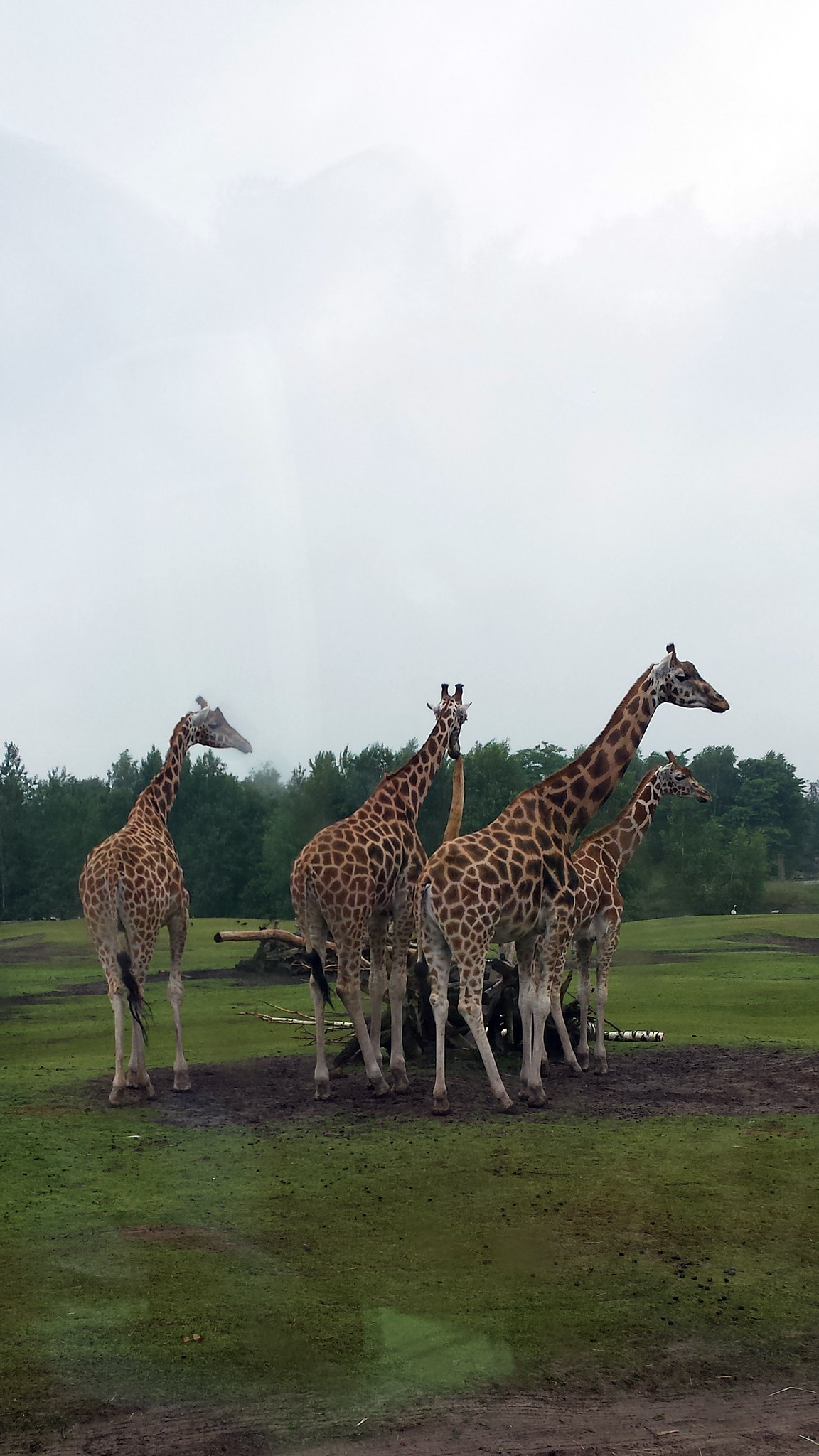In this detailed portrait-oriented photograph taken from inside a vehicle at a zoo or park, five giraffes stand prominently against a gray, overcast sky. The landscape features short green grass interspersed with churned-up patches of muddy earth, suggesting it has been recently raining. In the foreground, some dirt is visible, and the distant horizon showcases a line of tall green trees. A small tree limb or log lies on a slight hill in the background. The giraffes, bearing beige coats with distinctive brown markings of various shapes, are mostly grouped together with three huddled closely and one standing slightly apart. Among them, a shorter giraffe, possibly a baby, stands out next to an adult. Most of the giraffes gaze to the right, while one seems to look directly at the photographer. Reflecting the zoo environment, the picture captures the faint reflection of the photographer's arm and jacket in the vehicle window, subtly integrating the observer into the scene.